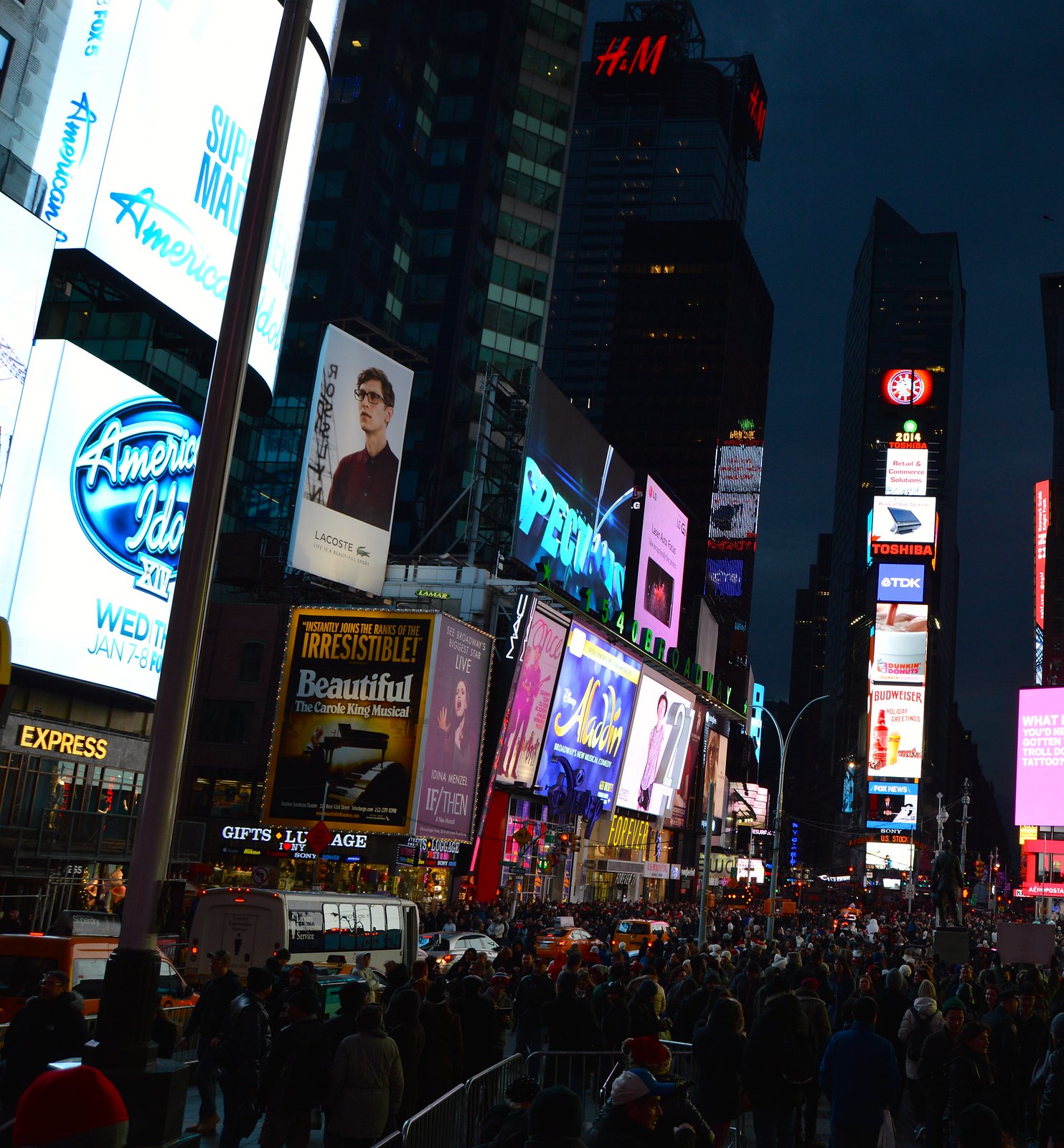This photograph captures a bustling evening scene in Times Square, New York City. The crowded street is teeming with pedestrians and vehicles, including a bus, a van, and several taxis and cars, all ensnared in bumper-to-bumper traffic. The surrounding skyscrapers are adorned with vibrant, neon-lit billboards advertising a variety of products and events. Notable signs include those for Toshiba, TDK, Budweiser, American Idol, Aladdin, Forever 21, and the Carole King musical "Beautiful." The famous New Year's Rockin' Eve location is recognizable by its distinctive flatiron-type building in the background. The sky is a deep blue, hinting at the encroaching night, while the bright lights from the billboards illuminate the throngs of people walking below. The scene is a quintessential snapshot of the energetic and iconic atmosphere of Times Square.